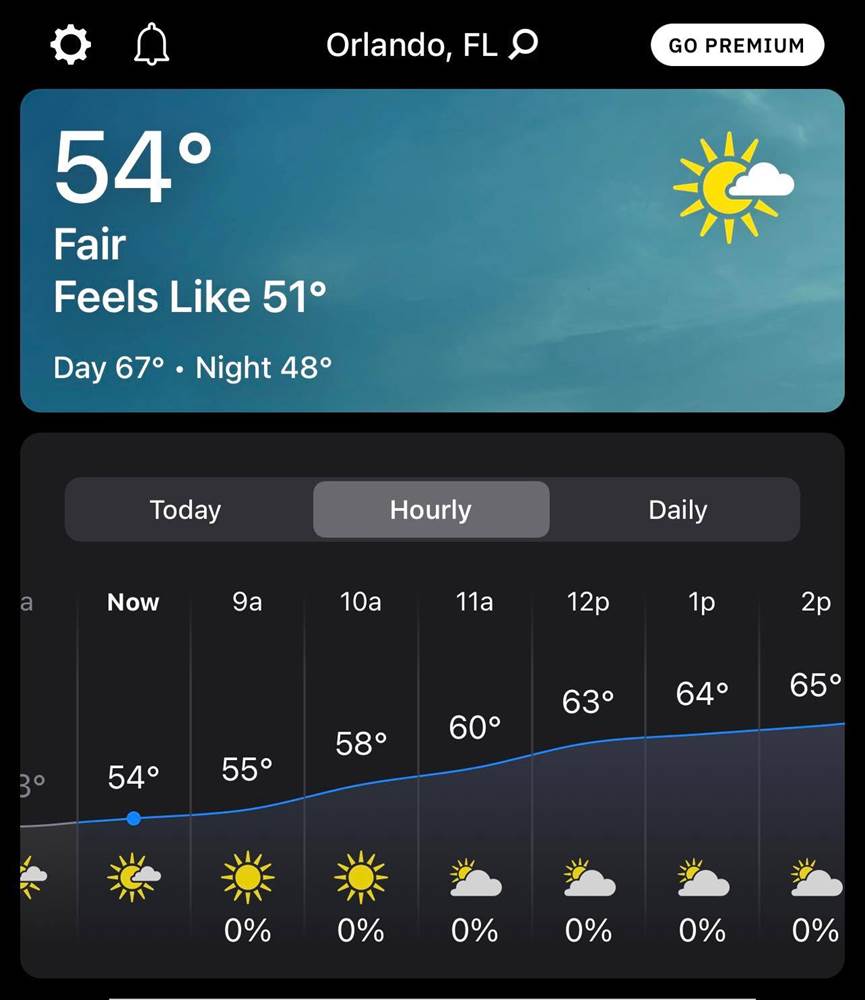Here is a comprehensive screenshot of a mobile weather application set against a black background. In the upper left corner, white icons for a settings cogwheel and a notification bell are prominently displayed. Centrally positioned at the top, "Orlando, FL" is shown with an adjacent magnifying glass icon indicating a search function. At the top right, a white oval-shaped button featuring black text invites users to "Go Premium."

Directly below, a blue background resembling a clear sky indicates the current weather conditions: "54 degrees, fair," with a "feels like" temperature of 51 degrees. Additional information includes a daytime high of 67 degrees and a nighttime low of 48 degrees, accompanied by a cheerful yellow sun partially obscured by a cloud icon.

Beneath this, navigation options for viewing "today," "hourly," and "daily" forecasts are available, with "hourly" currently highlighted. The detailed hourly forecast lists temperatures and weather conditions for the upcoming hours as follows:
- Now: 54 degrees
- 9 a.m.: 55 degrees
- 10 a.m.: 58 degrees
- 11 a.m.: 60 degrees
- 12 p.m.: 63 degrees
- 1 p.m.: 64 degrees
- 2 p.m.: 65 degrees

Each hour is accompanied by a weather icon, with a 0% chance of precipitation indicated at the bottom. The weather icons depict conditions ranging from sunny to partly cloudy skies.